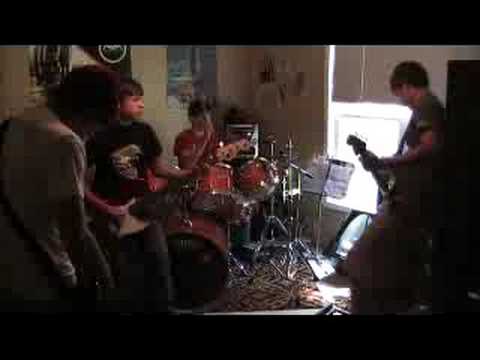The image depicts a blurry, digital photograph of a four-member band playing in a small, crowded bedroom. The dominant colors in the image are black and red, with additional accents of white, blue, and orange. Positioned in the corner of the room is a boy in a red shirt, energetically playing a red drum set placed on a rug. To his immediate left stands a boy in a black shirt and jeans, engaged with an electric guitar. Next to him, with his back against the wall, another boy in a white shirt strums an electric guitar. The fourth boy, leaning against a cabinet, attentively looks at sheet music on a music stand while playing his electric guitar. The room features a window on the far wall, which is slightly open, and scattered posters adorn the space, contributing to the cozy, intimate atmosphere of the spontaneous jam session. Despite the pixelation preventing clear views of their faces, the essence of youthful enthusiasm and camaraderie among the band members is evident.